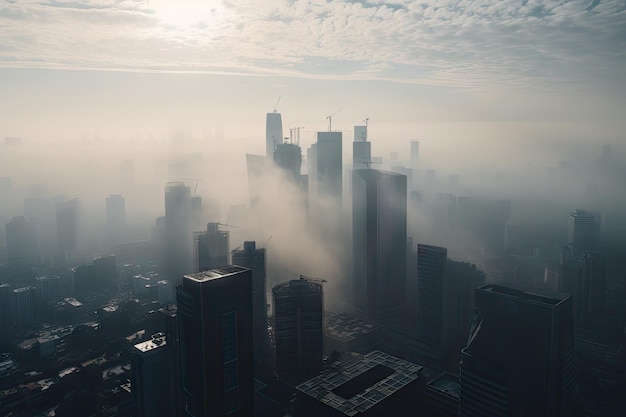The image depicts a sprawling, major metropolitan city distinguished by its numerous towering skyscrapers, some of which are undergoing construction or renovations as evidenced by the cranes perched atop them. The perspective appears to be from a high vantage point, offering a sweeping view of the city's skyline, characterized by high-rises of varying heights. The scene is cloaked in a dense, fog-like smog that obscures the lower parts of the buildings and gives a silhouetted appearance to the cityscape. The sky above is relatively clear with scattered white clouds, and the early morning sun or bright midday light filters through, illuminating the upper reaches of the skyline. The overall visual is somewhat monochromatic, with the fog lending a muted, almost eerie ambiance to the city, which remains nondescript and mysterious due to the lack of visible street details or recognizable landmarks.